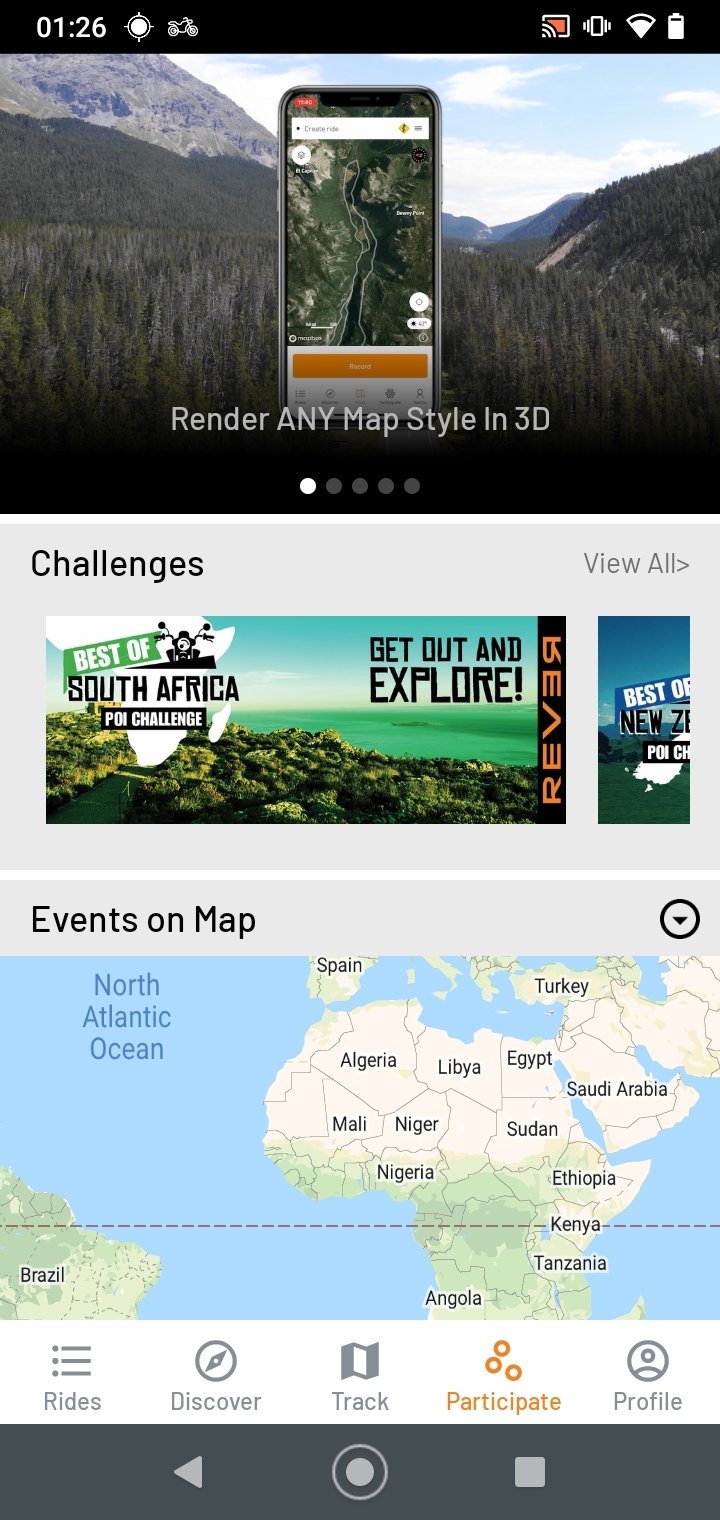The image described appears to be a complex interface, possibly from a digital application or website. Here's a cleaned and detailed caption:

---

The interface features a variety of elements:

1. **Header:**
    - At the very top, there is a black bar displaying the time "01:26."
    - A white circular icon with an outer ring, featuring small tips at the top and bottom. Within the circle, there's a white, indistinct squiggly symbol.

2. **Main Area:**
    - A section resembling a screen with a white rectangle containing a smaller red rectangle. On the bottom left, a Wi-Fi symbol is visible.
    - Adjacent is another rectangle with small triangles on the sides, resembling Wi-Fi or signal strength indicators.
    - Below these elements, an image of mountains is displayed.
    - In the background, there's a telephone displaying a road map.
    - A heading underneath reads "Render any map style in 3D."

3. **Middle Section:**
    - A series of circles: one white followed by four gray circles.
    - Below this is a gray rectangle with the text "Challenges" on the left and "View All" with a right-pointing arrow on the right.
    - A scenic picture in the corner labeled "Best of South Africa" with an illegible black rectangle.
    - Underneath, the text "Get out and explore."

4. **Promotions:**
    - A tall black rectangle with orange letters.
    - An image captioned "Best of..." indicating new content, which is partly cut off, featuring a blue top and green bottom.

5. **Additional Features:**
    - Another gray rectangle labeled "Events on Map" on the left, with a circle and downward-pointing triangle on the right.
    - Below is a map section.
    - Beneath the map are three vertically aligned sets of three dots and dashes.
    - Various labeled icons:
        - "Rides" with associated icon.
        - A circle with a central icon labeled "Discover."
        - A waving flag icon with the text "Track."
        - Three orange-outline circles labeled "Participate."
        - A profile icon within a circle, labeled "Profile."
    - A gray rectangle features a lighter gray left-pointing triangle, and a light gray outer circle with an inner circle and a square.

This detailed layout suggests a user interface designed for navigation and activities, possibly within a mapping or travel application.